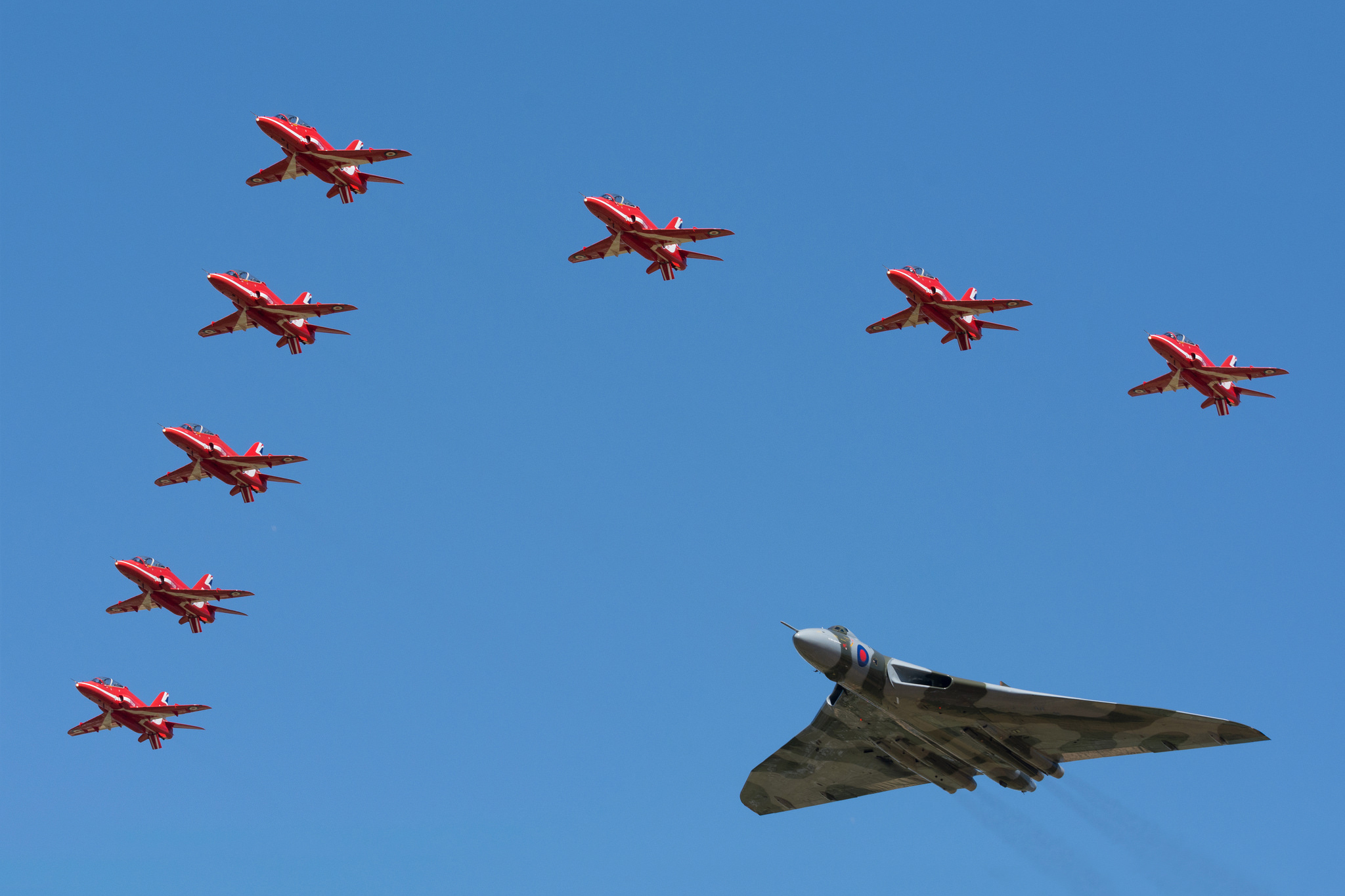The photograph captures a squadron of military air force planes soaring through a brilliant, cloudless blue sky. The primary focus is on eight red and white fighter jets arranged in a precise V formation, with four planes on each side of the lead aircraft that heads toward the upper left corner of the image. Below and slightly trailing this V formation is a larger, modern fighter jet, sporting a desert camouflage design. This aircraft features a V-shaped fixed wing, distinguishing it from the older straight-wing planes above. The image conveys a sense of ceremonial display, with the striking contrast of the older, red jets against the more contemporary camouflaged plane highlighting a blend of aviation history and modern technology.